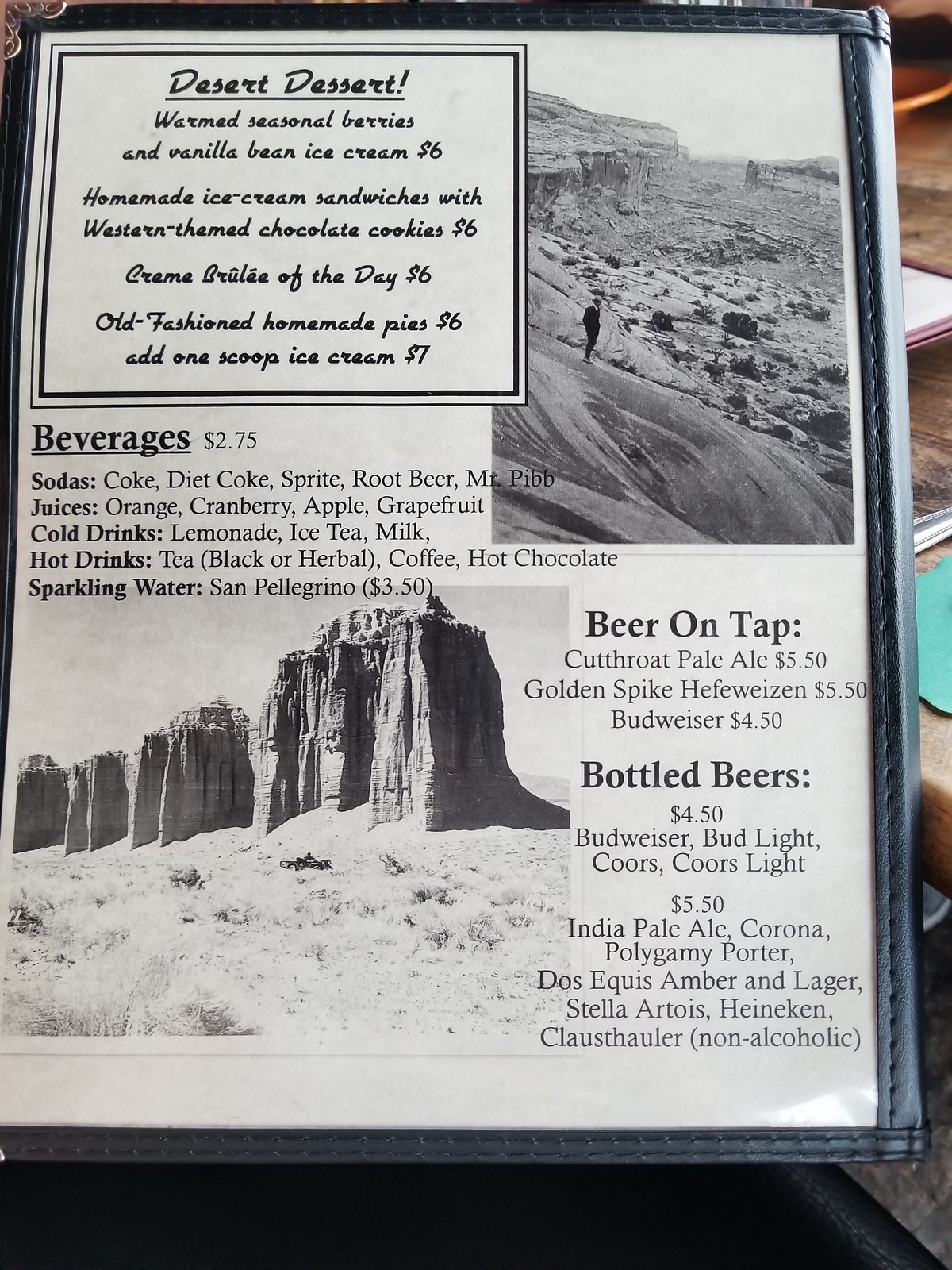In the photograph, a restaurant menu is encased in a sturdy, clear plastic cover, which is commonly used to protect menus. Towards the far right of the image, a wooden table is partially visible, adorned with place settings that include a fork and possibly a knife.

The prominently white menu features a few images depicting rugged terrain, contributing to its thematic design. At the top of the menu, there is a highlighted white square bordered in black. The menu's text is presented in black, drawing attention to its offerings.

Listed under "Desert Dessert," the options include:
- Warmed seasonal berries with vanilla bean ice cream for $6.
- Homemade ice cream sandwiches featuring Western-themed chocolate cookies, also for $6.
- Cream brulee of the day, priced at $6.
- Old-fashioned homemade pies for $6, with an option to add a scoop of ice cream for an additional dollar, totaling $7.

Below the desserts section, the menu details beverages:
- Sodas, juices, cold drinks, and hot drinks are priced at $2.75 each.
- Sparkling water, specifically San Pellegrino, is listed at $3.50.

The menu continues with a selection of beers, available both on tap and in bottles, catering to a variety of tastes.